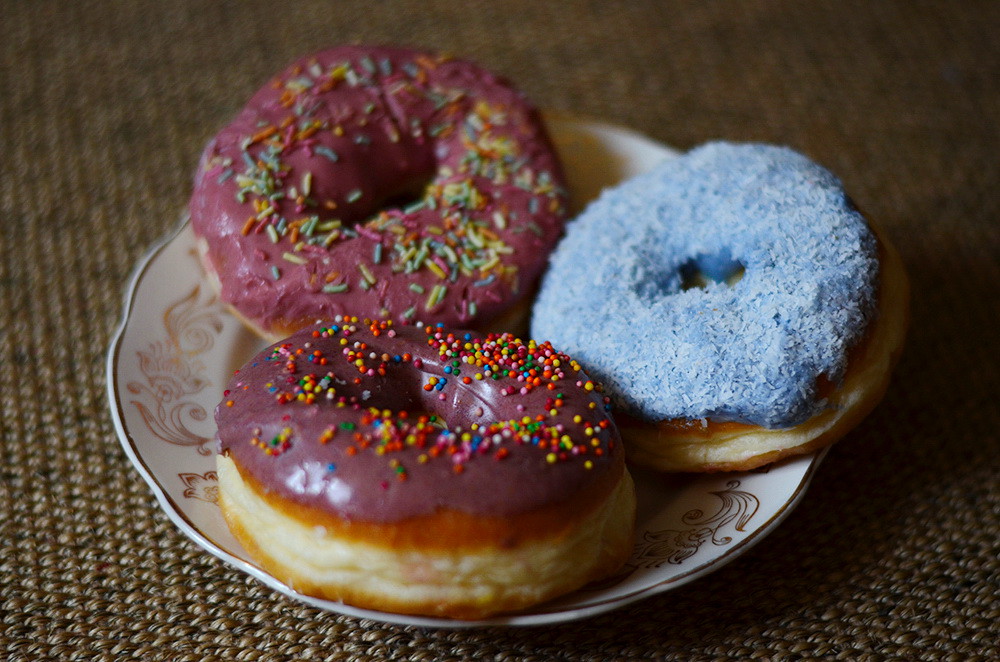This is a close-up photograph of three donuts arranged on an ornate, small plate that features delicate gold filigree around the edges and scalloped outlines, sitting on what appears to be a textured surface, possibly a carpet or table. Each donut, all seemingly bite-sized, is distinguished by its colorful icing and sprinkles. The first donut is adorned with pink frosting and topped with long, multicolored sprinkles. The second donut features purple icing with round, tiny, multicolored ball-shaped sprinkles. The third donut exhibits a blue frosting with white shavings, likely coconut, adding a textured appearance. The intricately designed plate enhances the visual appeal of the vibrant, moist-looking donuts, making them stand out in the photograph.